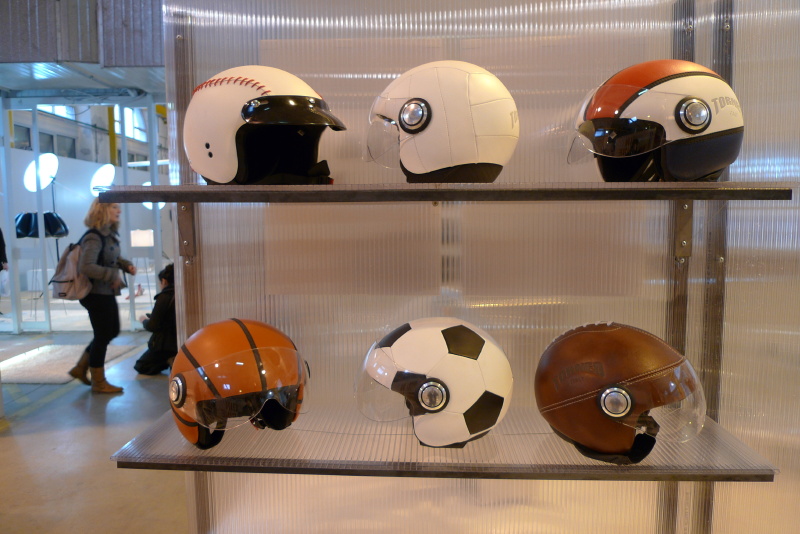This photograph presents a meticulous display of six sports-themed helmets arranged on two floating wooden-framed acrylic shelves with ridged backgrounds. Each shelf holds three helmets, neatly aligned, transforming the space into a visually captivating presentation, ideal for a retail store or museum setting.

On the top shelf, the helmet on the left is designed to mimic a baseball, featuring a white base adorned with a distinctive row of red stitching. The middle helmet resembles a volleyball, characterized by its white surface with interlacing seams creating a dynamic pattern. Completing the top row, the helmet on the right showcases an orangish-red stripe bordered in black, reminiscent of a racing theme.

The bottom shelf continues the sports motif with an orange and black basketball-themed helmet on the left. The central helmet on this row is marked by white hexagons and black pentagons, perfectly emulating a soccer ball. Lastly, the rightmost helmet on the bottom shelf resembles a leather football, complete with textural brown finish and white stitching details.

In the background, the setting provides further context with its polished concrete floor and an ambiguous environment that could hint at a retail space, exhibition, or even a photo shoot. Amid the scene are various figures including a woman in a gray shirt, gray backpack, dark denim pants, and dark brown shoes, contributing to the sense of public space and human interaction. The overall composition and intricate helmet designs create a compelling visual study of sports culture and artistic design in everyday objects.